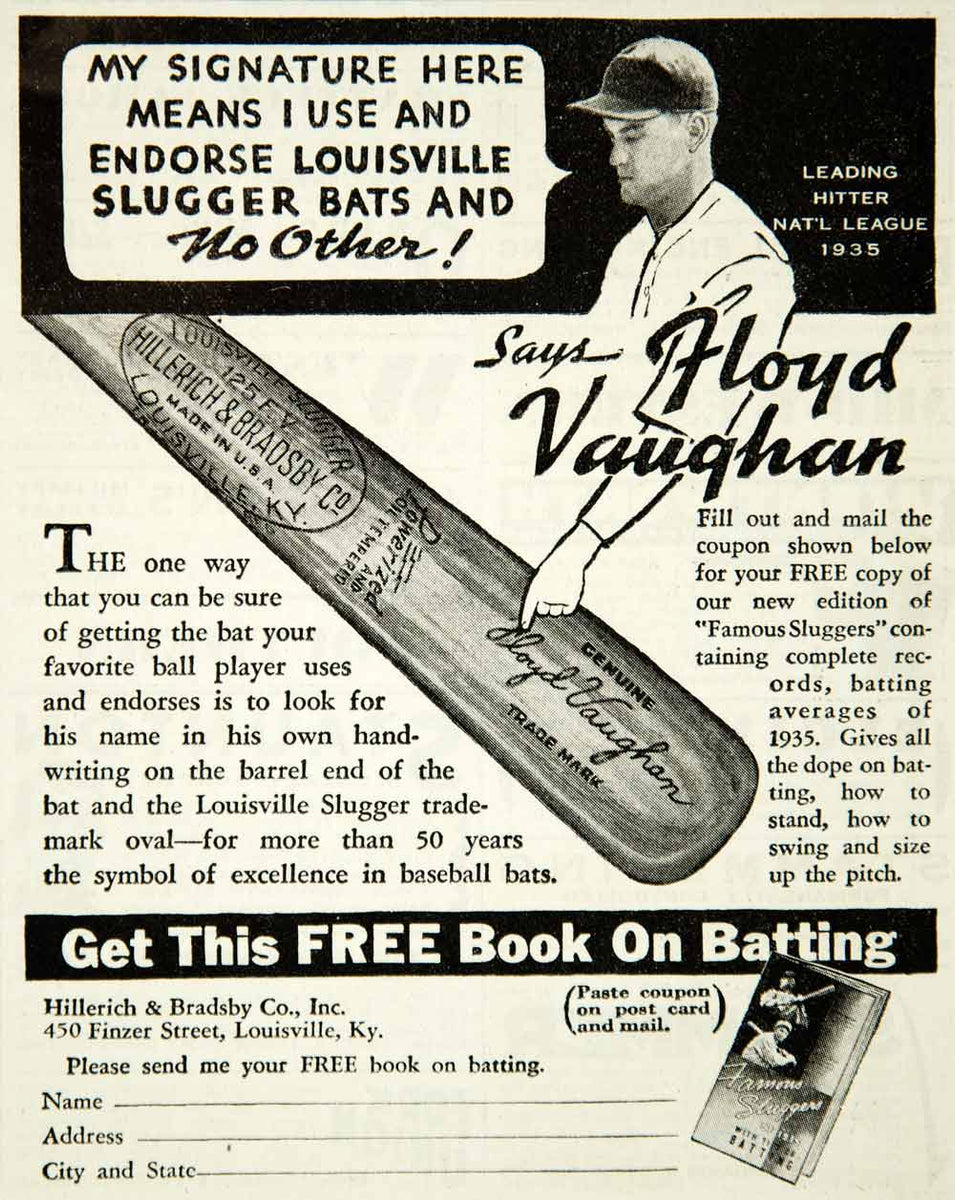The advertisement, reminiscent of an old, yellowed magazine print, features a black and white image predominantly highlighted by a black background at the top quarter. In this section, a baseball player, Lloyd Vaughan—identified by the text to the right reading "Leading Hitter, National League, 1935"— is depicted wearing a baseball hat and uniform. A thought bubble near his face contains the text, "My signature here means I use and endorse Louisville Slugger Bats and no other!"

An arm extends from this section, pointing towards a bat displayed diagonally on the bottom right, inscribed with details such as "Louisville Slugger," "Hillerich and Bradsbury Company," "Made in USA," "125 FV," and "Louisville, Kentucky." Below, more text encourages readers to look for the player's signature on the barrel end of the bat to ensure they are getting the endorsed model.

At the bottom, the advertisement promotes a free book on batting with instructions to mail a coupon to Hillerich and Bradsbury Company, Inc., 450 Finster Street, Louisville, Kentucky, to receive a copy of "Famous Sluggers" containing batting records and tips from 1935.